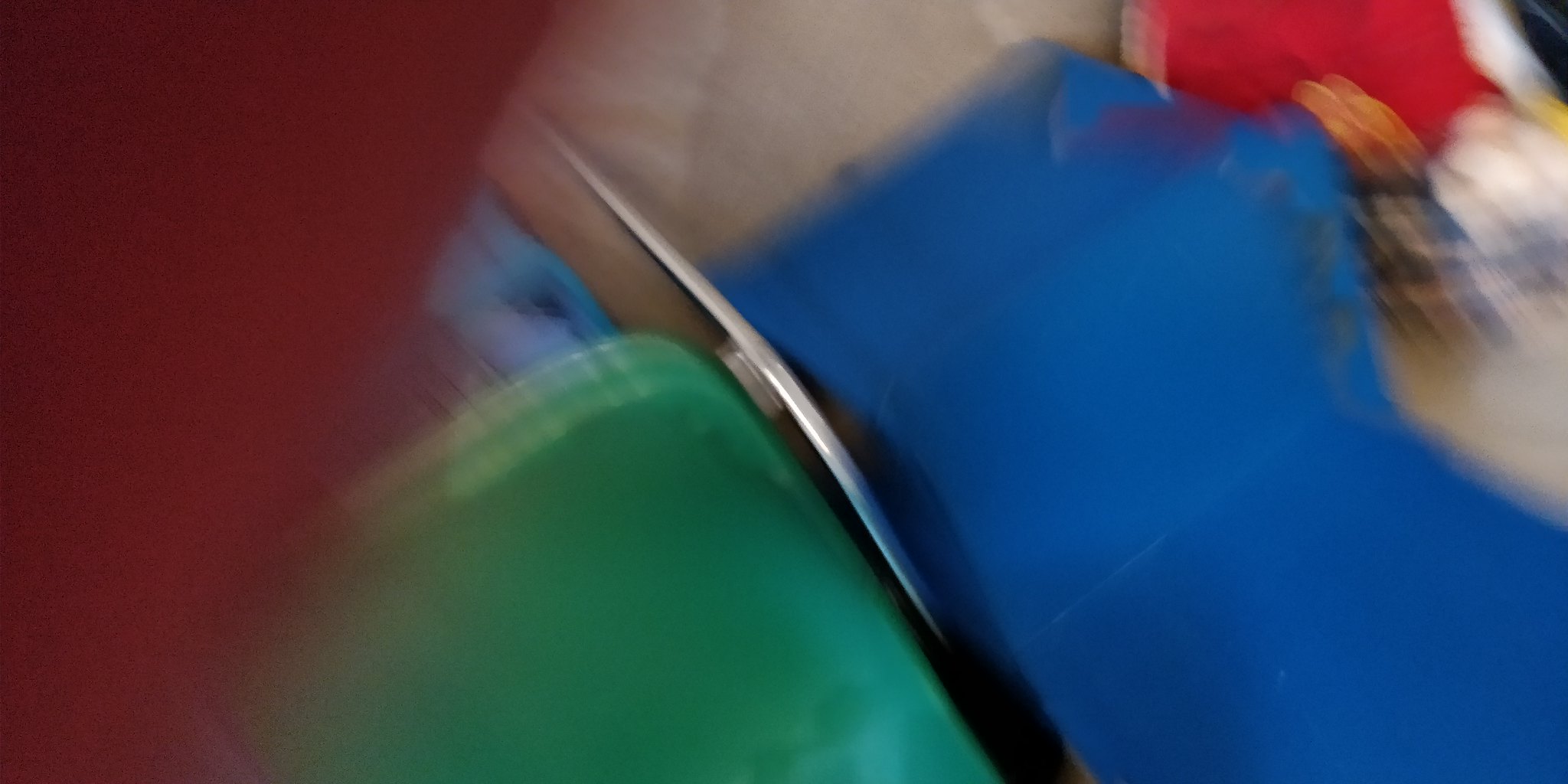This is an extremely blurry photograph, likely taken accidentally with a smartphone. The image is dominated by a flesh-toned blur, possibly a finger, which covers much of the top left corner, extending diagonally downward. Scattered across the blurred background, several objects can be vaguely identified: a green plastic chair with chrome legs, a bright blue chair or box, and various indistinguishable blobs of color including red fabric and blue plastic. In the upper right corner, a mix of red, white, and orange shapes can be seen, possibly a basket or fabric. The overall scene is too blurry to detail with precision, but it appears to depict a casual, cluttered area with several pieces of furniture.